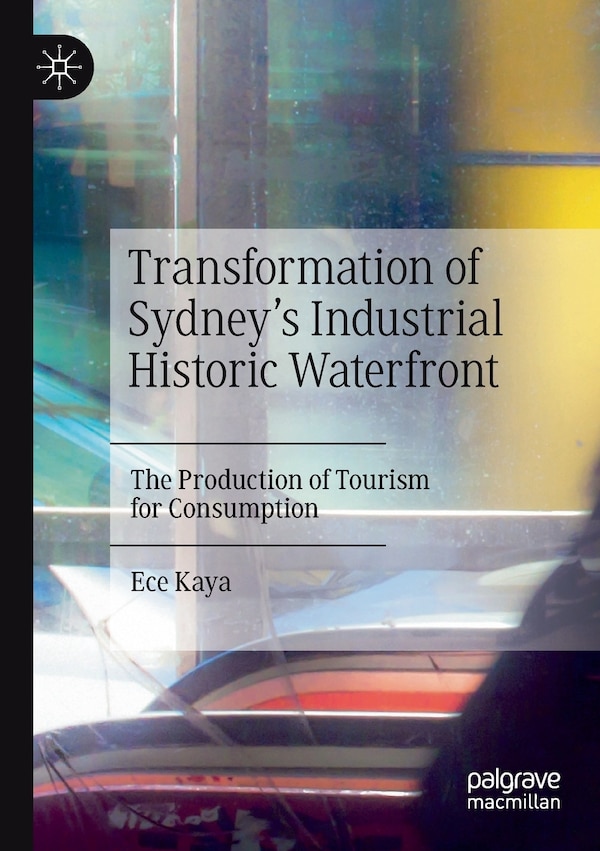The cover of the book "Transformation of Sydney's Industrial Historic Waterfront: The Production of Tourism for Consumption" by E.C. Kaya, published by Palgrave Macmillan, features a detailed photograph as its background. The photo appears to capture an urban scene, possibly depicting a station or an area undergoing renovation, with an escalator leading down to the tracks at its center. Behind the escalator, there is a wall with a pillar and floor-to-ceiling windows, which have an aqua and yellow hue. The text is placed within a central gray text box, with black font. Additionally, a distinct black border runs along the left edge of the cover. The publisher’s name, Palgrave Macmillan, is located in the bottom right corner in white text. Overall, the cover blends elements of modern construction with historic references, encapsulating the book's theme of urban transformation.